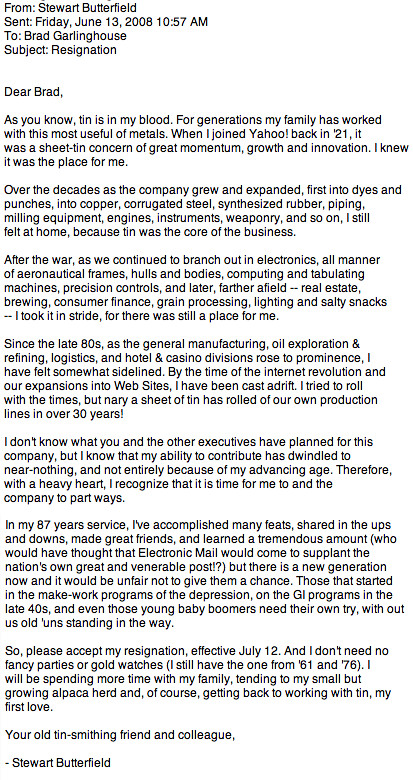The image is of an email on a white background with black text, titled as a resignation letter. Sent from Stuart Butterfield to Brad Garlinghouse on Friday, June 13, 2008, at 10:57 AM, the subject line reads "Resignation." The letter opens with "Dear Brad" and details Stuart's long-held passion for tin, a tradition in his family for generations. He joined Yahoo! in 1921 when it was a thriving sheet tin company known for its momentum, growth, and innovation. Over the decades, as the company expanded into various sectors such as dyes, punches, copper, corrugated steel, synthesized rubber, and more, he always found his place because tin remained central. However, as the company diversified into electronics, aeronautics, real estate, brewing, consumer finance, and beyond, Stuart began to feel sidelined, particularly since the late 1980s. Despite trying to adapt, he felt adrift by the time of the internet revolution as tin production ceased over 30 years ago. Acknowledging that his ability to contribute had diminished, he decided to resign effective July 12th. Stuart reminisces about his 87-year service, the evolution of communication through electronic mail, and emphasizes the importance of giving new generations a chance. He concludes by expressing his preference for no elaborate farewell events, mentioning his old gold watches from 1961 and 1976, and stating his intention to spend more time with family and his alpaca herd, and to return to tin-smithing. The letter is signed, "Your old tin-smithing friend and colleague, Stuart Butterfield."